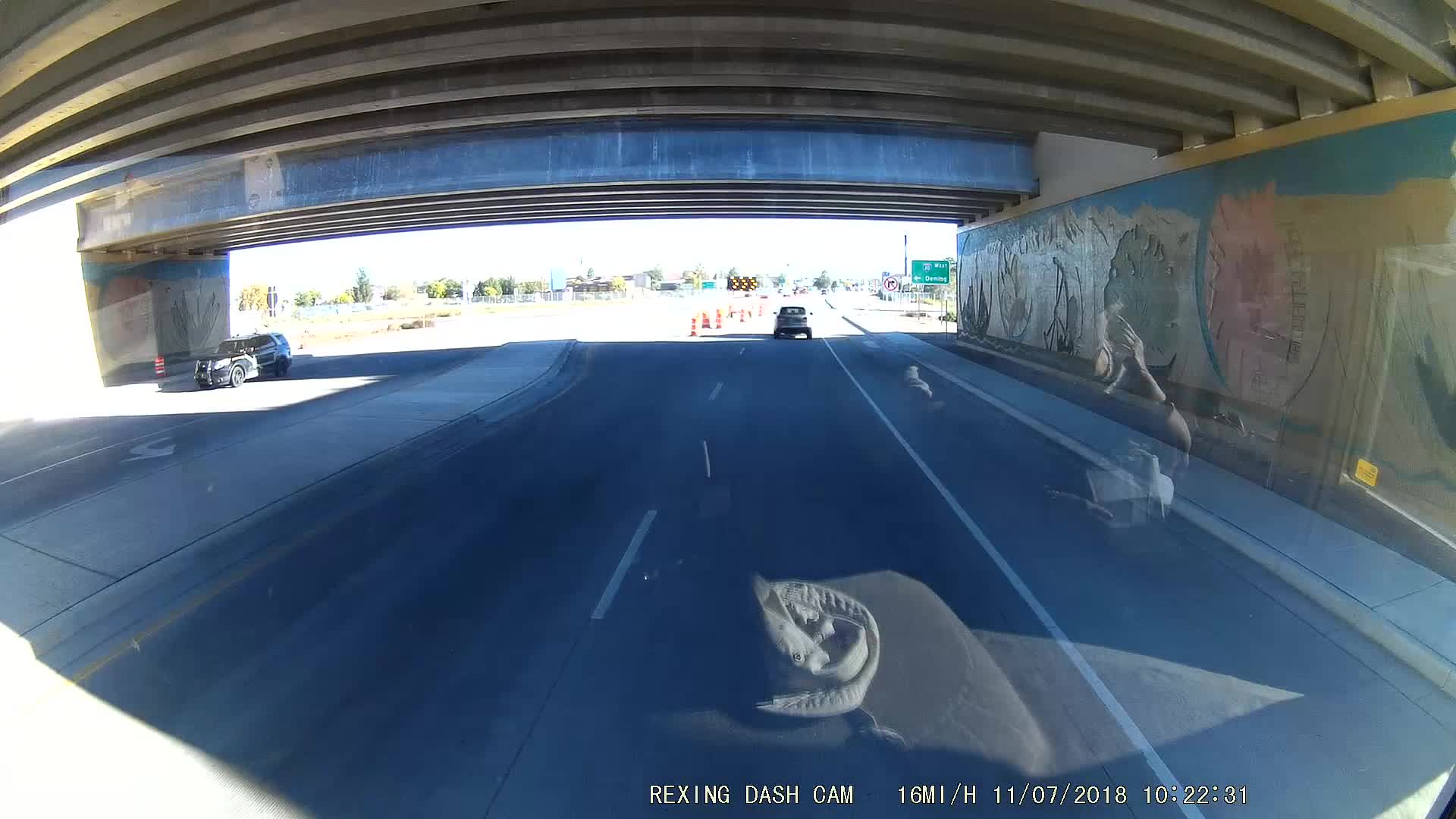The image is a color photograph taken from a dashcam, visible through the front windshield of a car. The bottom of the image is stamped with the text "REXING dashcam," along with the date "11-07-2018" and the time "10:22:31." In the foreground, a reflection of something white, possibly a tissue, is on the dashboard.

The scene captures a highway under a freeway overpass, characterized by massive concrete beams with gaps, indicating a divided highway with four lanes on each side. The underpass walls are adorned with murals featuring large faces, blue sky, and flowers, enhancing the urban aesthetic. A green highway sign, presumably with an interstate shield, is visible ahead.

Traffic is directed by orange cones, and an arrow suggests that the left lane is closed, guiding vehicles to the right. A concrete median separates the lanes from oncoming traffic, where a car with an open door appears stationary, possibly for photographing the murals. A car is visible farther ahead in the same lane as the dashcam vehicle. The background reveals a distant cityscape against a clear, sunny sky, suggesting a bright day. Some rubbish is noted on the floor of the underpass, contributing to the urban feel of the scene.